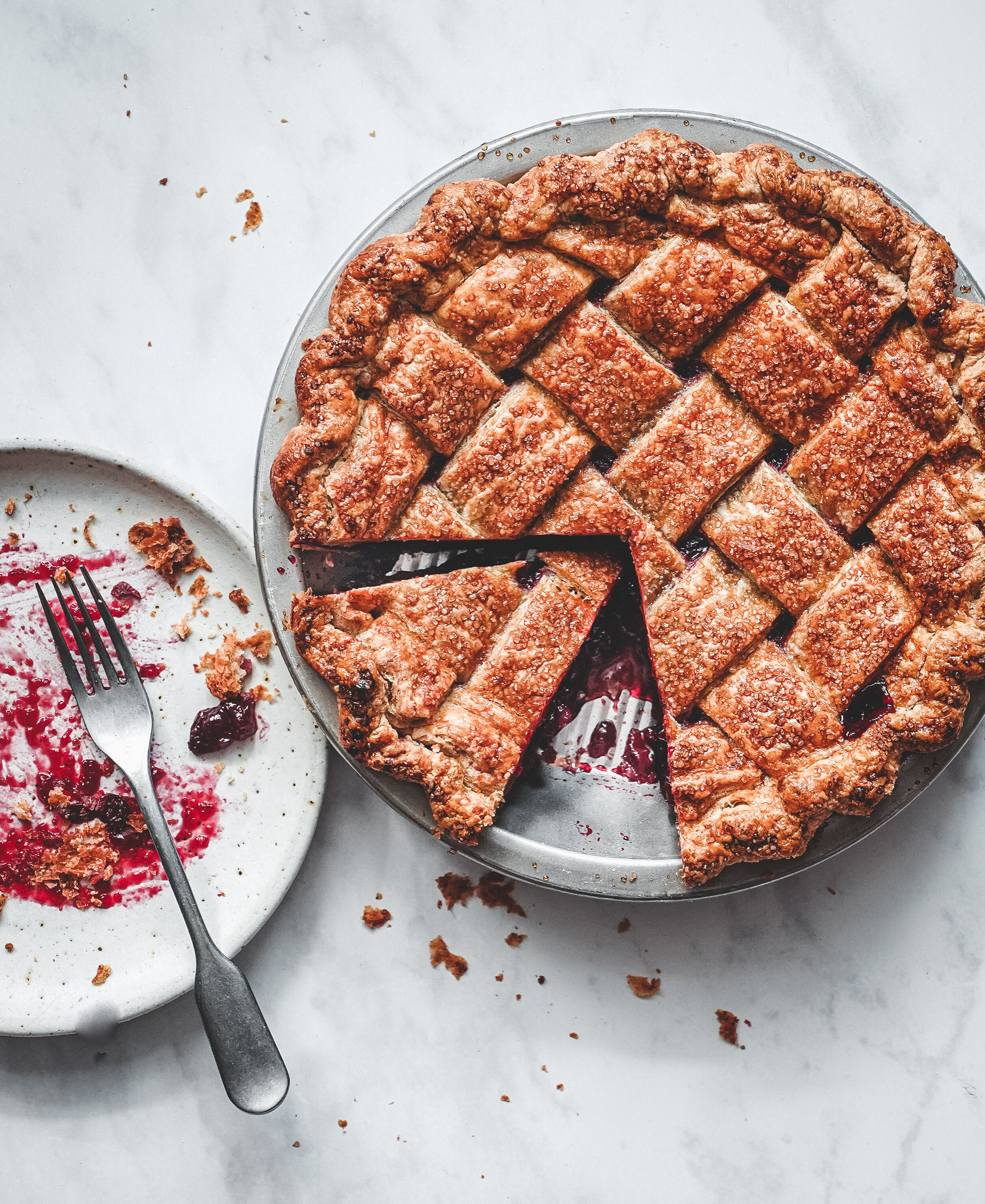This photograph, taken from a bird's eye view, showcases a cherry pie with a meticulously woven lattice crust, hinting at a possible light dusting of cinnamon on its golden-brown surface. The pie, occupying the right side of the image, is presented in a metal pie tin that rests on a pristine white marble table. Approximately a quarter of the pie is missing from the bottom left quadrant, with one slice completely removed and another cut but left in the pan, revealing the dark reddish filling typical of cherries. Adjacent to the pie tin on the left, a white plate displays the remnants of a enjoyed slice—noticeable cherry smears and scattered crumbs—alongside a silver fork that dangles off the plate's edge, suggesting someone didn't scrape off all of the delicious filling. The photograph is oriented vertically, emphasizing the detailed arrangement and aftermath of a delectable treat.